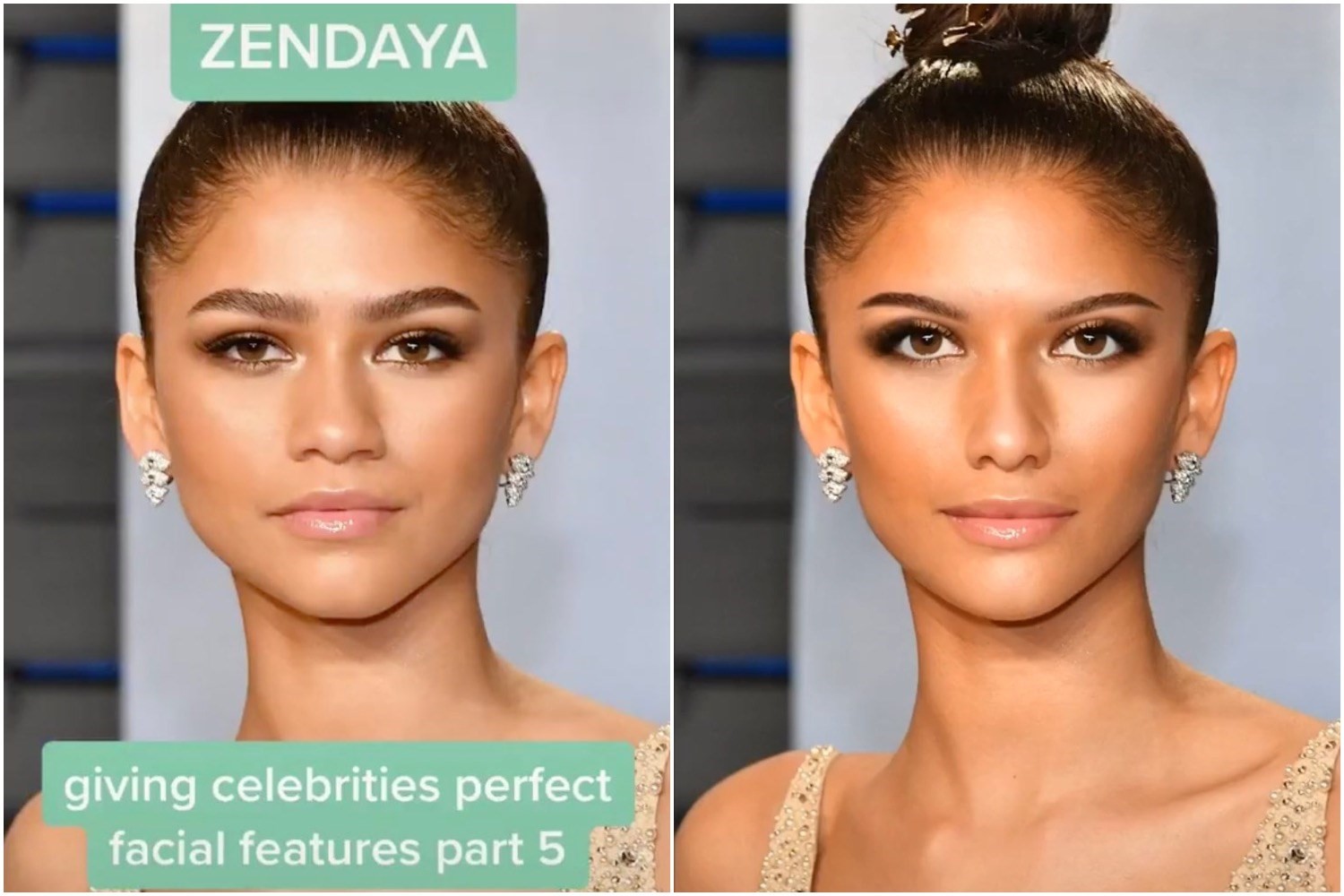The image is a side-by-side comparison featuring two photographs of the same girl, intended as part of a tutorial. On the left, the girl's face appears slightly tired, particularly around the eyes. This side is labeled with text reading "Zendaya, Giving Celebrities Perfect Facial Features Part 5." The right-hand image, in contrast, shows the same girl with noticeable enhancements: her eyes appear lifted, her eyebrows are arched and thinner, giving her a more refreshed and polished look. This transformation seems to be achieved through digital manipulation rather than actual makeup application, likely intended for a tutorial on a website or social media platform. While the edited right-hand image looks appealing, it also has an unnatural quality when compared to the more natural appearance on the left.